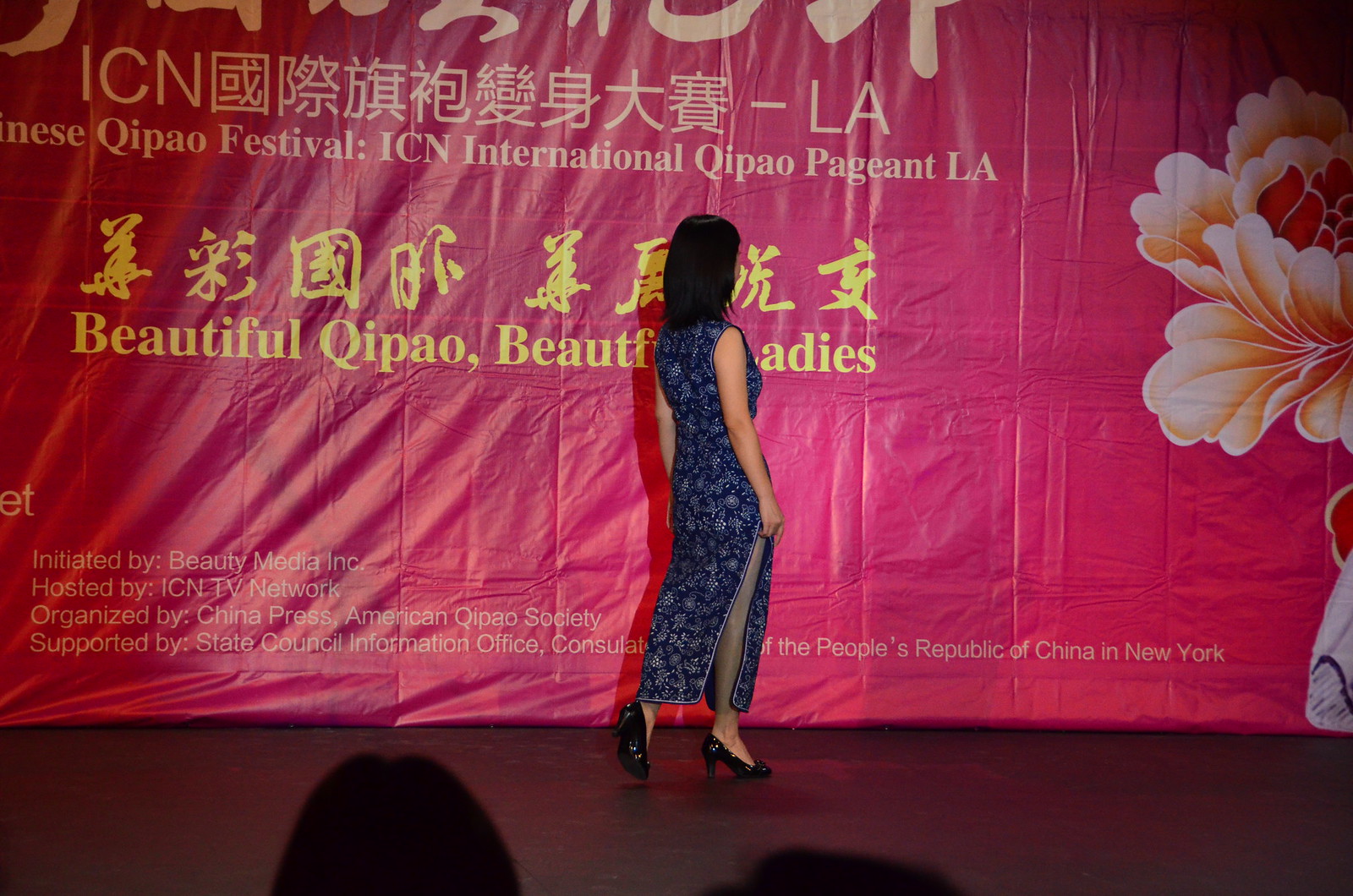This wide rectangular color photograph captures an Asian woman walking on a smooth, black stage. She has light skin and black hair, and she is wearing a striking, ankle-length blue qipao with white and silver floral patterns. The dress is form-fitting with an angular cut that reaches up to her thighs, which she is holding together. Her black high-heeled pumps shine under the stage lights. The woman’s back is somewhat to the camera, and she is facing a large, bright pink banner that swoops from the top edge and is adorned with an image of an orange and red flower on the right side. Silhouettes of audience members' heads are faintly visible at the bottom of the image. The banner behind her features yellow Chinese characters, and prominently displays the text "Beautiful Qipao, Beautiful Ladies" in yellow font. The rest of the banner has alternating Chinese and English text, mentioning event details such as "Initiated by Beautiful Media Incorporated" and "Hosted by ICN TV Network." The visible portion of the banner includes the text "Kapa'a Festival ICN International Kapa'a Pageant LA," along with other sponsor information in small white text.